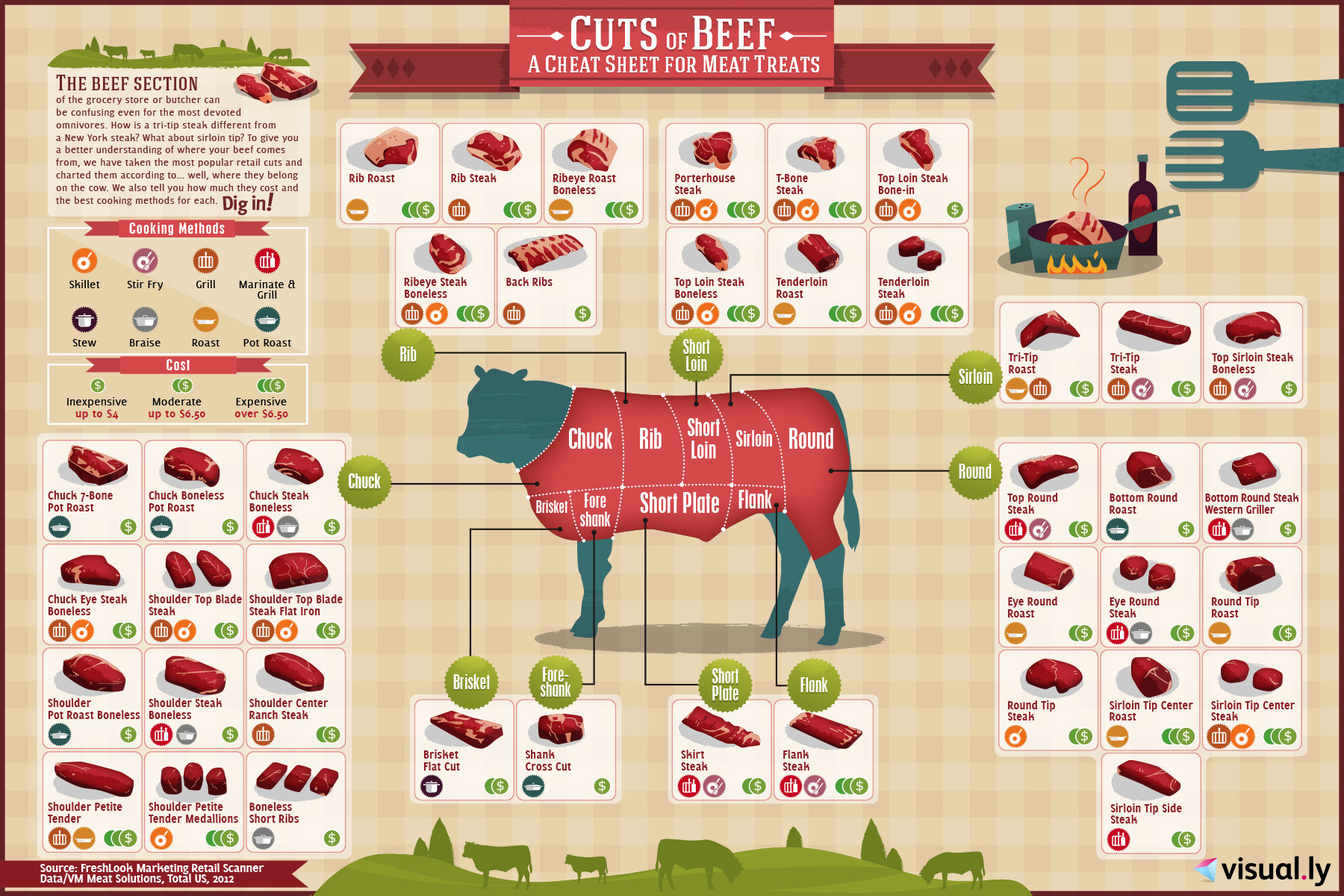In the photo, there is a large, visually appealing display detailing various cuts of beef. This informative exhibit is accentuated by a prominent red banner at the top that reads, "Cuts of Beef: A Cheat Sheet for Meat Treats." 

On the left side of the display, there is a paragraph titled "The Beef Section," providing an overview of beef types and qualities. Adjacent to this, a "Cooking Method" section lists different ways to prepare each cut, including skillet, stir-fry, grill, marinade, stew, braise, roast, and pot roast.

Below this, a cost indicator divides the cuts into categories such as inexpensive, moderate, and expensive. Following this, the display showcases cuts starting with pot roast, boneless steak, and going on to include pork shoulder, steak shoulder, and corner ranch steak, noting that the shoulder cut is the most expensive.

Central to the display is a detailed diagram of a cow, marking the locations of various cuts including brisket, chuck, short plate, flank, round, sirloin, short loin, and rib. The overall presentation is educational, offering a comprehensive guide to understanding beef cuts and their uses.